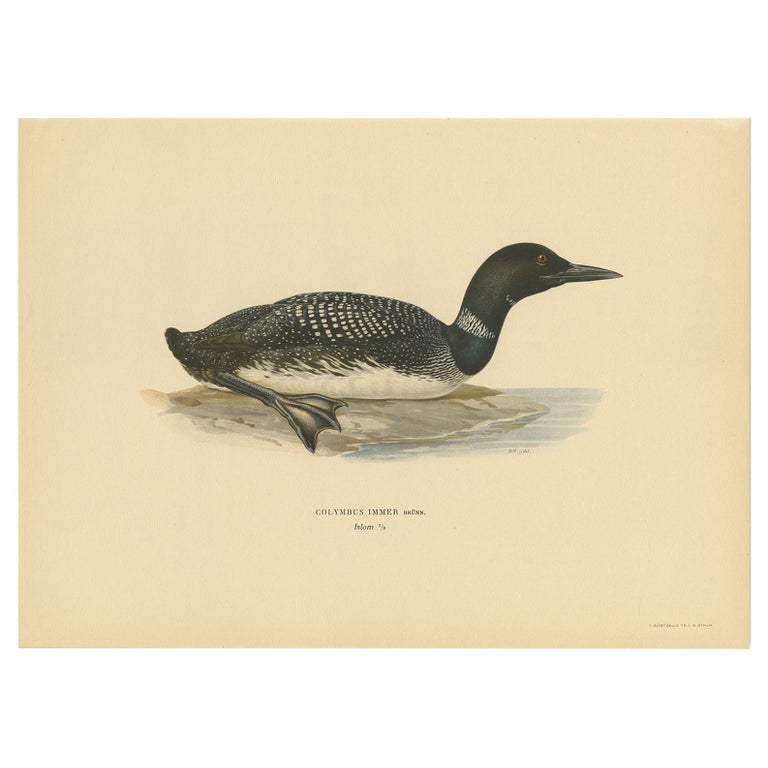The horizontal rectangular image on aged, yellow parchment paper features a detailed vintage illustration of a duck resting near the waterline. The duck is centered in the composition and depicted in full color with meticulous attention to detail. Its head is black with a metallic green sheen, and it has a pointed gray beak. A distinctive white band encircles its neck. The duck's back is adorned with dark brownish-gray feathers patterned with rows of tiny white dots, and its belly is white. Its black webbed feet are tucked under its body, suggesting it is poised to re-enter the water. Faint text in a foreign language is visible beneath the illustration. The background behind the duck is a light brownish or creamy yellow shade, likely due to the paper aging over time. This vintage piece captures the serene moment of the waterfowl resting and embodies a classic artistic style.